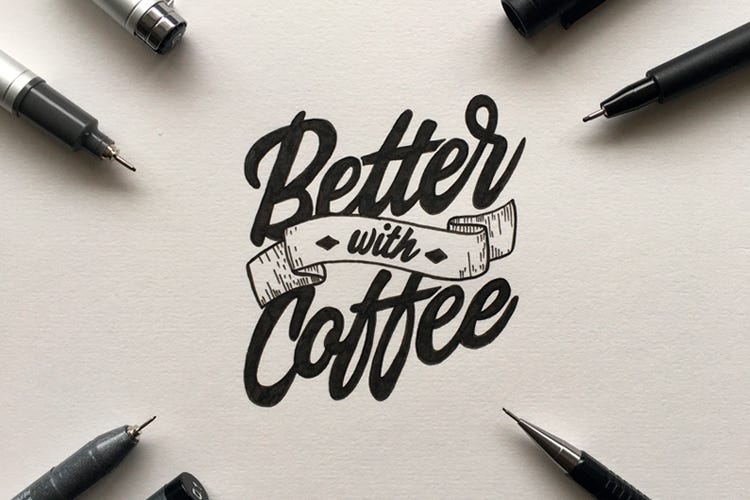The image features a color slide or graphic ideal for a PowerPoint presentation, set against a white background. Central to the composition is the phrase "Better With Coffee," crafted in a stylish and elegant cursive font that gives the impression of hand-written text. The words "Better" and "Coffee" are rendered in a large, bold black script, while the word "With" is displayed in a smaller font, flanked by two diamond symbols and encased in a ribbon-like design that resembles a tape measure marked with tiny lines. Encircling the central text are seven black ink pens with silver tips, meticulously arranged with two pens positioned at the bottom, two at the top left, two more at the top right, and one at the bottom right, creating a balanced and visually appealing frame for the script.